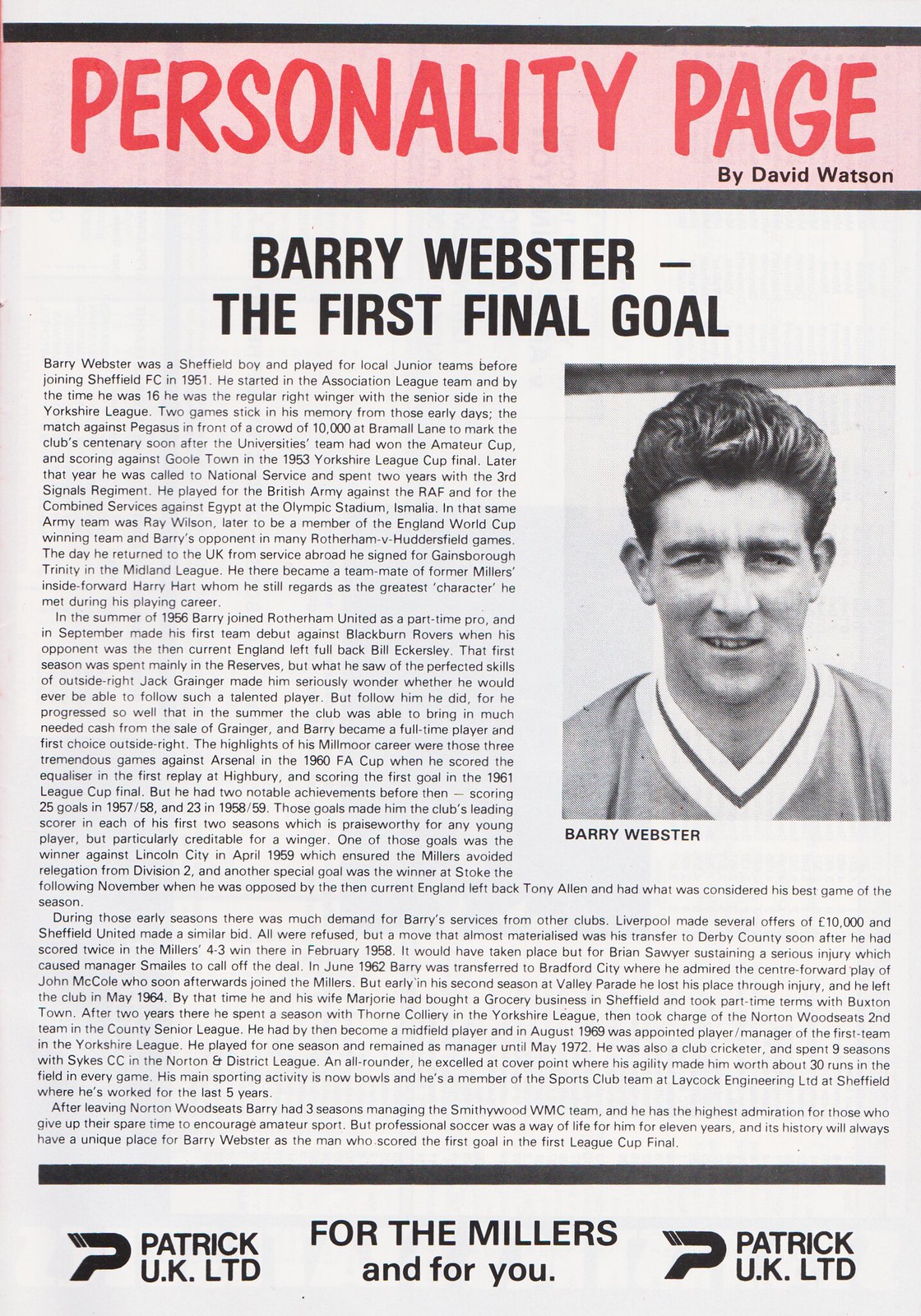This image is a photo of a magazine article page titled "Personality Page" by David Watson, prominently displayed in large red capital letters on a pink horizontal strip at the top. Below this, the title of the article, "Barry Webster - The First Final Goal," is presented in bold black capital letters. The article itself spans three to four paragraphs, detailing Barry Webster's biography, including who he played for and his statistics. On the right side of the page is a black-and-white photograph of Barry Webster, who appears to be wearing a v-neck soccer jersey. Below his photograph is a caption with his name. At the bottom of the page, there are various logos and text, with the words "For the Millers and for you," as well as mentions of "Patrick UK LTD" on both the left and right sides.